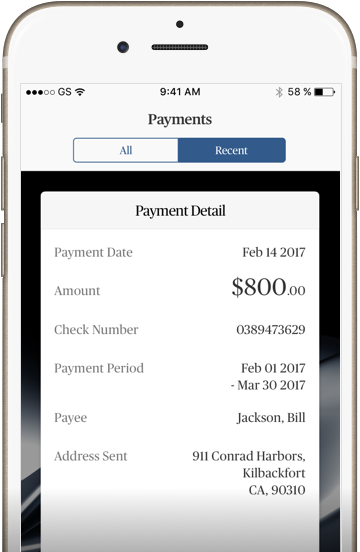This image is a detailed screenshot taken on a cell phone, showcasing an interface related to payment details. The cell phone's outline is visible, including the volume buttons on the left and the power button on the right. At the top center of the phone, there is a circular area for the camera, below which lies an oblong speaker grille.

In the top-left corner of the screenshot, there are five horizontal dots, the first three are black, and the last two are white. Adjacent to the right, the letters "GS" are displayed, followed by upward-facing triangular bars indicating signal strength. The status bar further shows the time as 9:41 a.m. Moving rightward, there is a Bluetooth icon, a "58%" battery percentage indicator, and a battery icon showing it is 58% charged.

In the middle of the image, the screen prominently displays the word "Payments" in blue. Below this, there are two buttons: a white button with the word "All" in blue on the left, and a blue button with the word "Recent" in white on the right.

The lower part of the screenshot elaborately details a payment summary, starting with the title "Payment Detail" in black text. Below that, the "Payment Date" is listed in gray on the left as "February 14, 2017" in darker gray. This pattern continues as follows:

- "Amount" in light gray on the left, with "$800" in darker gray on the right.
- "Check Number" in light gray on the left, with "0389473629" in darker gray on the right.
- "Payment Period" in light gray on the left, with "February 1, 2017" in darker gray on the right.
- "Payee" in light gray on the left, with "Jackson, Bill" in darker gray on the right.
- "Address Sent" in light gray on the left, with "911 Conrad Harbors, Killback Fort, CA 90310" in darker gray on the right.